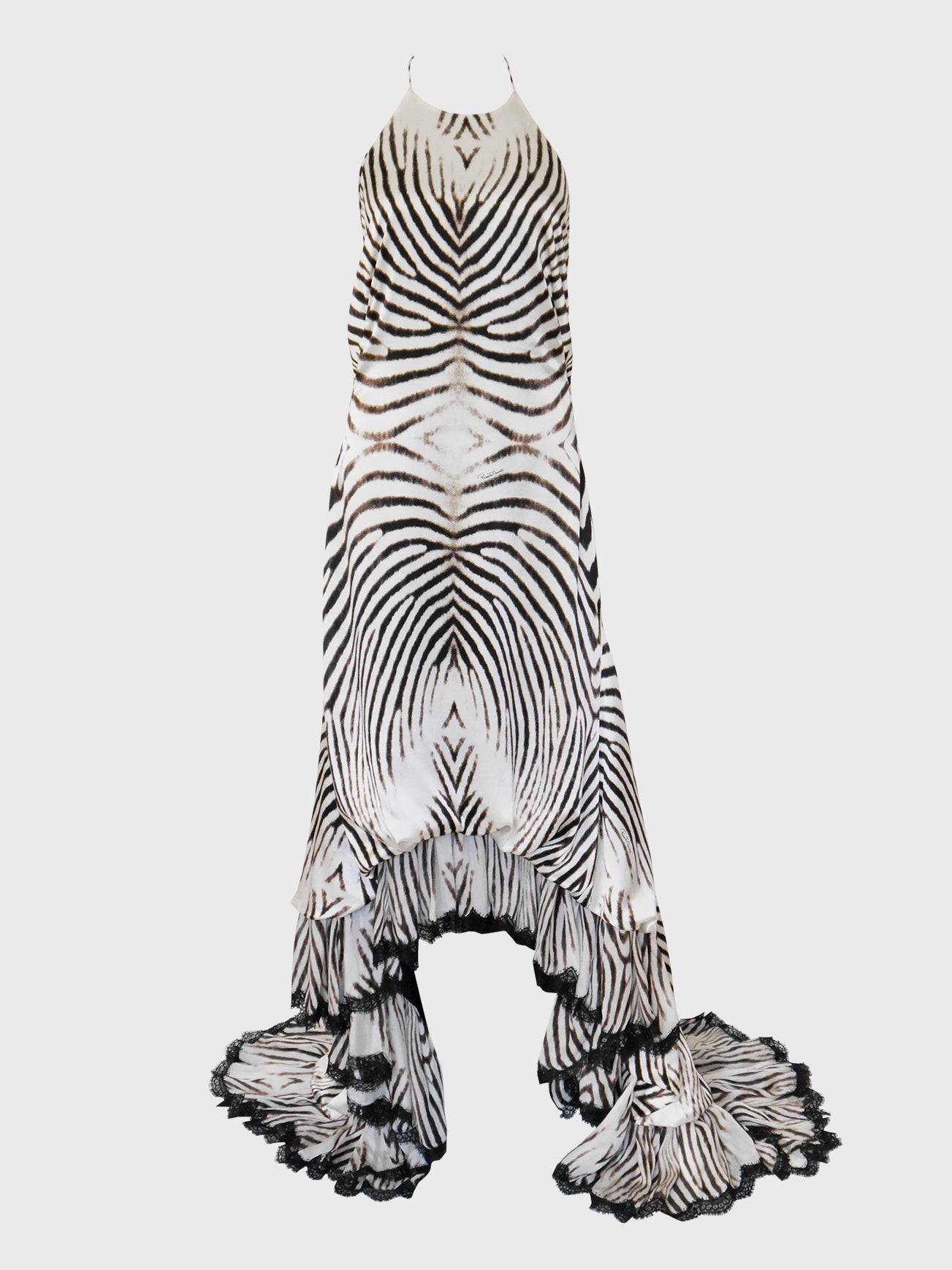The photograph captures an elegant black and white dress with an intricate zebra print pattern. The dress features thin straps and a loop that wraps around the neck, creating a halter-style neckline. Flowing gracefully down, the dress is composed of multiple layers that cascade to the ground, each layer outlined with delicate black lace detailing. The pattern is mostly symmetrical, with striking stripes that center to form a diamond shape at the torso. The edges of the dress flare out as they drape downward, resembling a curtain with black frayed or lace-bordered edges. The background is a stark, light grey, emphasizing the dress as the focal point, which stands upright as if worn, yet remains suspended in mid-air.